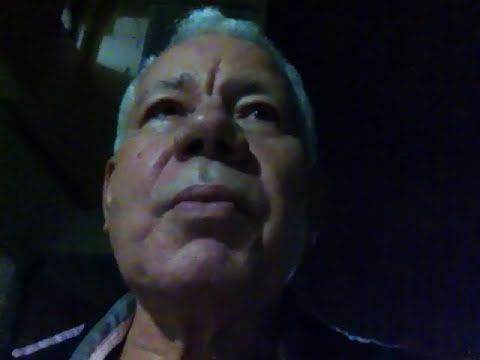This close-up photo captures an older white man with silver-gray hair styled short. His serious, unsmiling face is set against a dark, almost black background. The man’s wide nose and full lips are prominent, and his deep furrowed brow adds to his intense expression. He has a distinctive mustache but is otherwise clean-shaven. His dark eyes are gazing slightly upward, hinting that the camera is positioned just below him, allowing a partial view into his nostrils. His face occupies most of the frame, showing a hint of redness, especially on the left cheek and chin. He wears a shirt featuring a mix of colors including dark blue, light blue, yellow, and a white stripe, but the details are somewhat fuzzy due to low light or focus. There is no text in the photograph, and the background remains undefined, adding to the image's somber and contemplative mood.